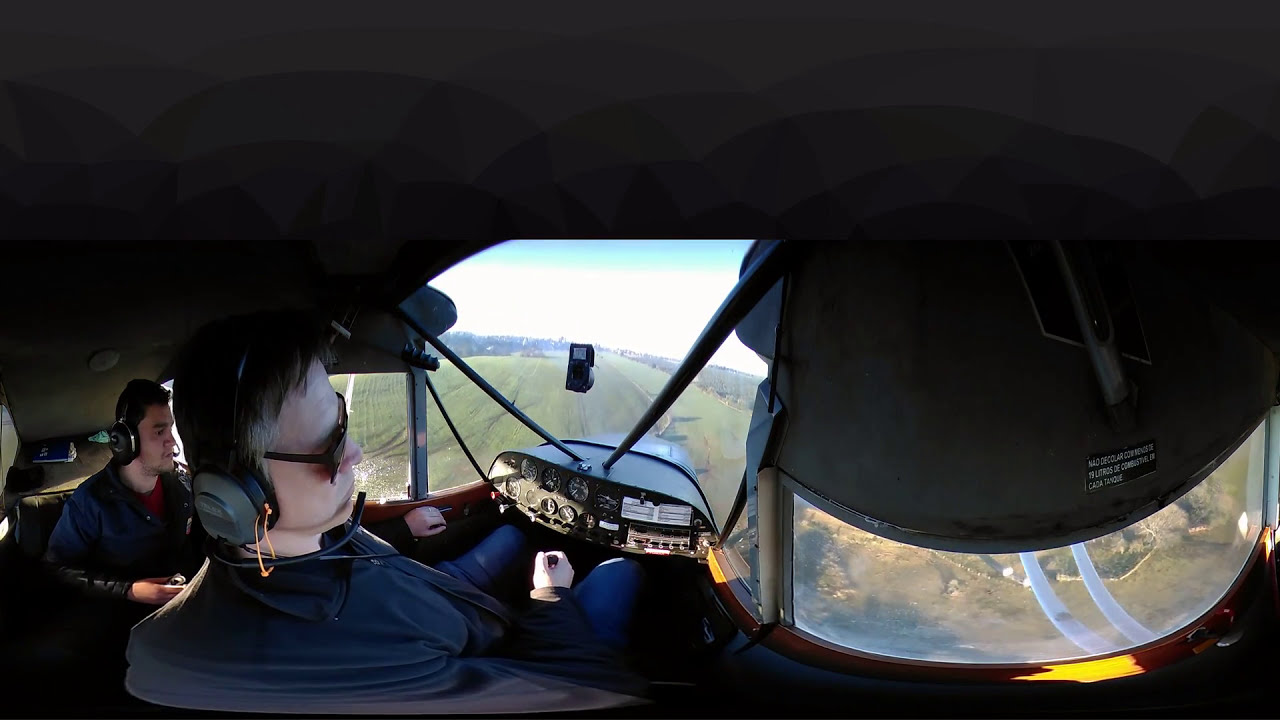This image is a panoramic view of the cramped cockpit of a small airplane, possibly a single-engine aircraft, showing some distortion due to the narrow space. The photograph centers around the pilot, a white male in his early forties with black hair peppered with white on the sides. He is wearing sunglasses and over-the-ear headphones, along with a blue zip-up windbreaker and Levi's blue jeans. The pilot's right hand grips the control stick situated between his legs, guiding the plane toward a green grassy runway visible through the windshield, indicating an imminent landing.

To the left of the pilot, another white male, also in his forties with dark hair, is seated. He, too, wears over-the-ear headphones and a similar blue zip-up sweatshirt. A split-screen section in the lower left corner of the image also reveals this second individual more clearly.

The cockpit features a small cluster of dials and controls on the left side of the picture, emphasizing the aircraft's operational complexity. Through the windows, the lush, green countryside spreads below, indicating the rural landscape they are flying over.